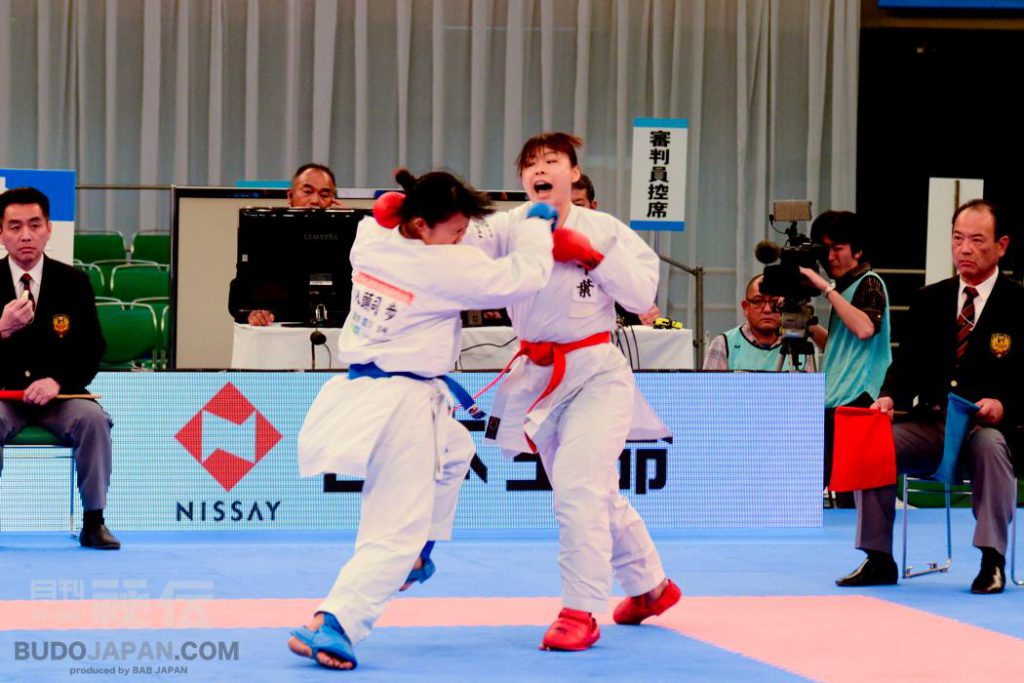In this highly detailed image of a martial arts sparring match, set within a professional competition context likely in Japan, two young Asian women, possibly in their late teens or early 20s, are engaged in a fierce karate bout. The competitor on the right, identified by her red belt, gloves, and slippers, is captured mid-strike, her right fist aimed at her opponent with her mouth open, possibly shouting or grunting. Her challenger on the left dons a blue belt, gloves, and slippers, mirroring the standardized white karate outfit worn by both.

The scene unfolds on a blue mat with a pink border, emphasizing the formal setting of the event. A panel of officials, dressed in black suits and ties, can be seen in the background, each holding red and blue flags to indicate round winners. Additional elements that suggest the event's authenticity and location include a camerawoman in a blue vest filming the match and several pieces of Asian script, likely Japanese, adorning the walls and a poster partially obscured by the fighters. The bottom of the image features a web address, budojapan.com, credited to BAB Japan, further anchoring the scene as a martial arts competition in Japan.